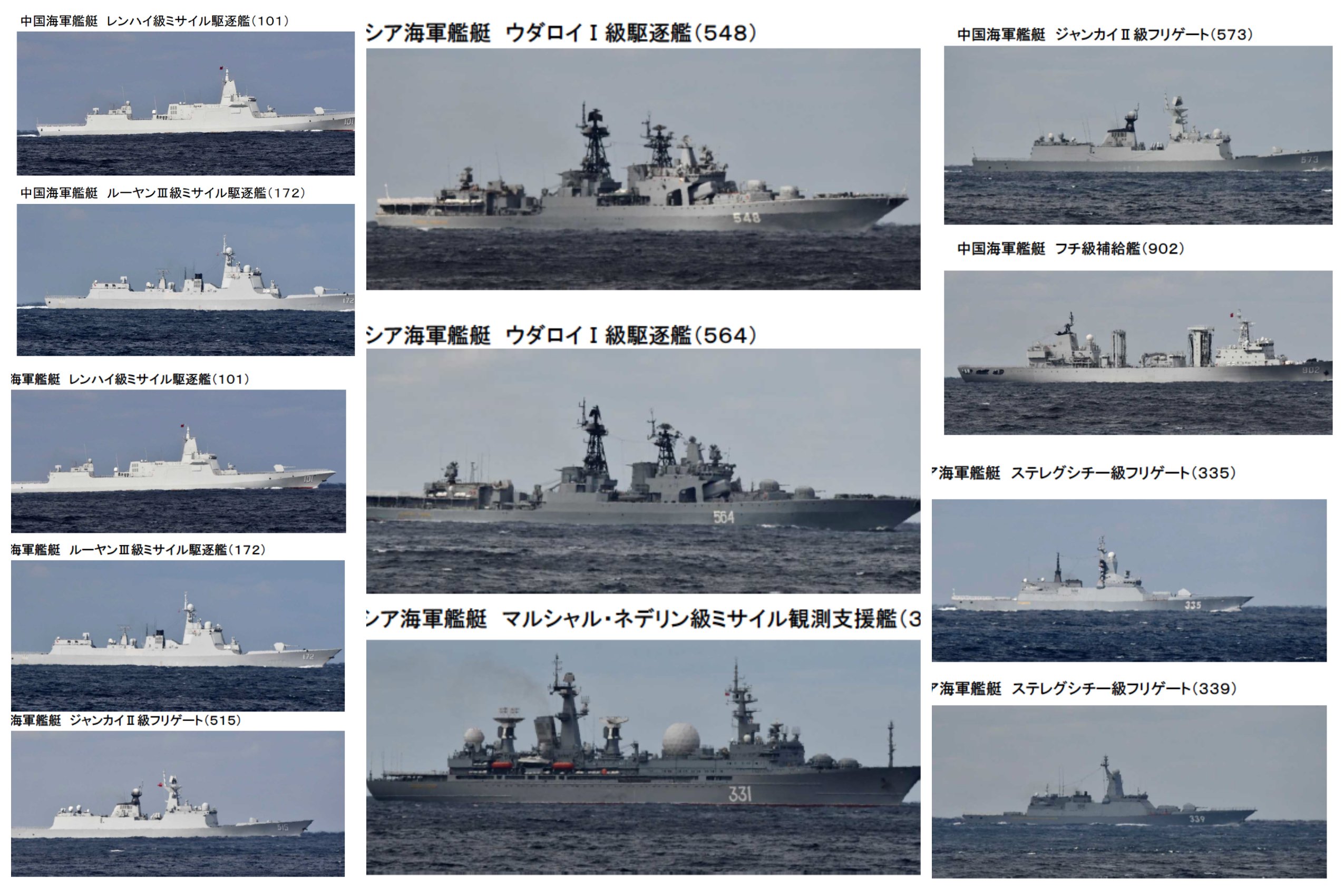The image features a detailed chart of various military ships, organized neatly into three distinct columns and four rows. Each ship is meticulously illustrated, with all the images set against a maritime backdrop.

In the first column, there are five ships, all painted similarly and sharing a general resemblance, with slight variations such as differences in antennae and a noticeably larger deck gun on the ship at the bottom. The second column contains three ships, all uniform in appearance with a similar gray color scheme and white numbers on their hulls; the top ship is numbered 548, the middle one 564, and the bottom one 331, each differing slightly in the equipment situated on their upper decks. The final column presents four ships, which are mostly alike in shape but display varying paint schemes; notably, the top two ships in this column are uniformly gray.

Each image within the chart is labeled, though some labels are in oriental writing, making them difficult to interpret. The smaller images and detailed labels contribute to the technical aesthetic of this chart, underscoring its focus on the precise and comparative visual presentation of military ships.